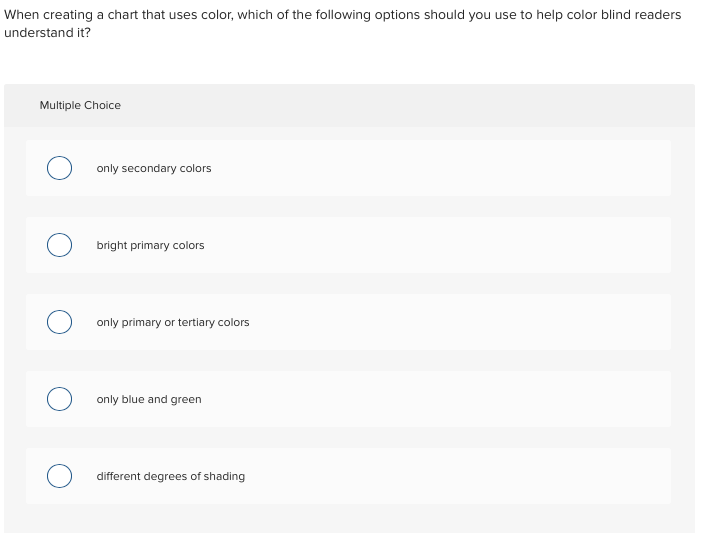This image portrays a digital test screen displaying a multiple-choice question designed to assess knowledge regarding the creation of accessible charts for colorblind readers. The screen features a sleek and modern layout with a sturdy contrast between its elements. The question, written in a black or dark gray font on a white background, asks: "When creating a chart that uses color, which of the following options should you use to help colorblind readers understand it?"

Below the question, the interface is segmented into a structured box with a dark gray band at the top, labeled "Multiple Choice" in clear, legible text. The main section of the box is filled with a slightly lighter gray color, creating a subtle yet effective differentiation.

Within this main area, five individual answer boxes are presented, each in an even lighter shade of gray. These answers are:
1. Only secondary colors.
2. Bright primary colors.
3. Only primary or tertiary colors.
4. Only blue and green.
5. Different degrees of shading.

Each answer option is accompanied by a clickable white circle with a blue outline on its left side, allowing the test-taker to select their response. 

The overall design ensures readability and accessibility while guiding the user through the test.